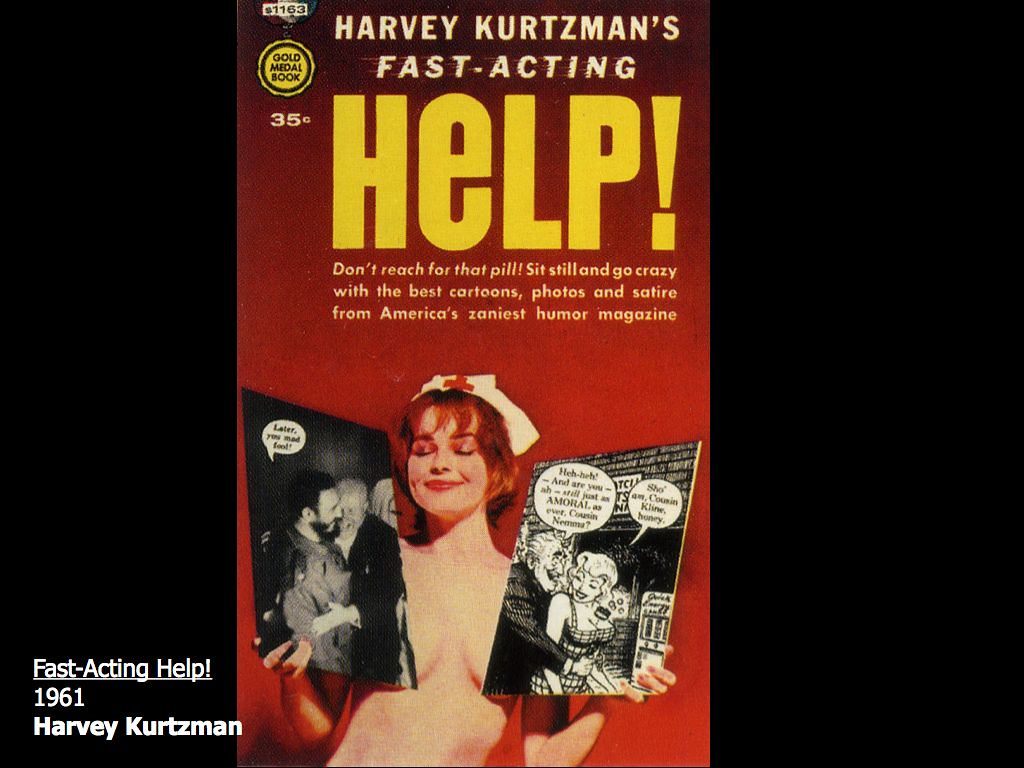The image depicts a vintage book cover from 1961, featuring a striking red background with the top section labeled "S1163, Gold Medal Book, 35 cents" in gold medallion style. Dominating the center third of the cover are bold yellow letters spelling out "Harvey Kurtzman's Best Acting Help!" accompanied by the tagline, "Don't reach for that pill. Sit still and go crazy with the best cartoons, photos, and satire from America’s zaniest humor magazine." The focal point is a woman, presumably an old-fashioned nurse, with red hair and a white nurse hat adorned with a red cross. She is smiling with her eyes closed while holding two black-and-white cartoon images over her breasts, giving her a playful and risqué appearance.